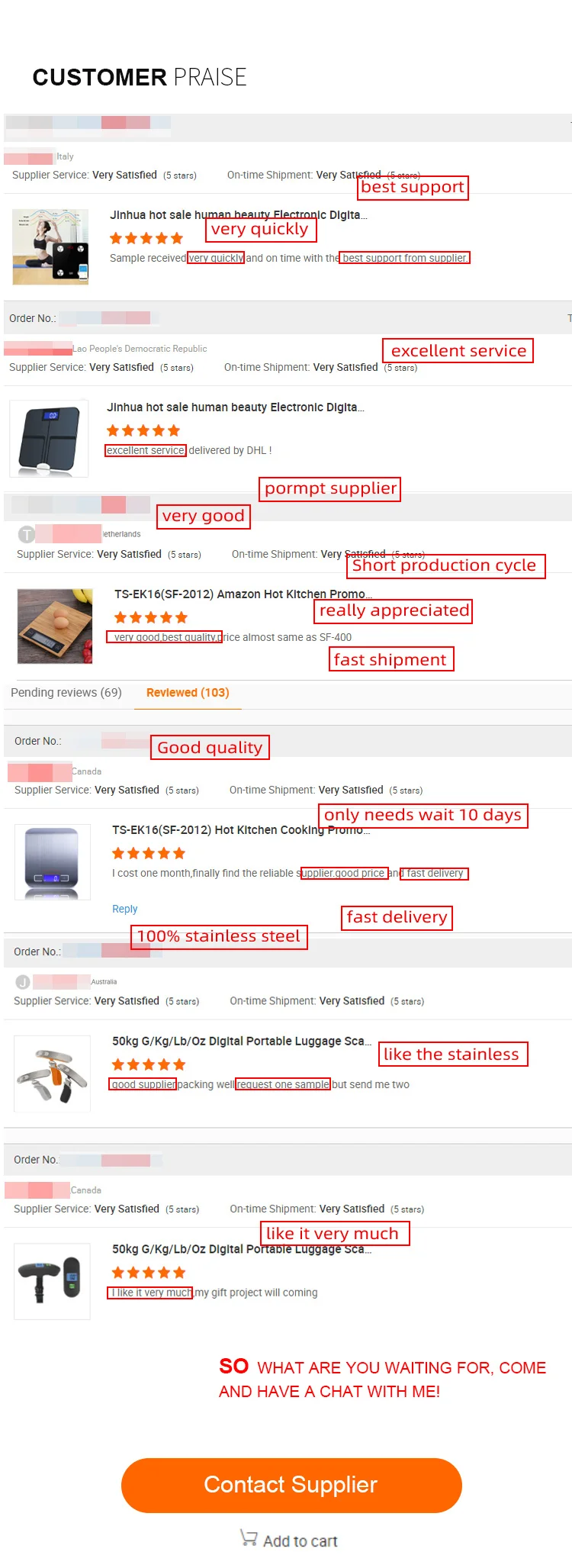The image showcases a storefront labeled "Customer Praise," characterized by a series of product listings accompanied by images and detailed descriptions. Each product is adorned with positive affirmations within red squares, highlighting accolades such as "Best Support," "Very Quickly," "Excellent Service," "Prompt to Supplier," and "Very Good." These commendations are prominently displayed next to each product, underscoring a consensus of high customer satisfaction.

The products range from electrical goods to everyday sales items, each clearly titled to denote its category. At the bottom of the image, a red banner extends a call to action: "SO, what are you waiting for? Come and have a chat with me." Beneath this, a prominent orange button encourages contacting the supplier, while another option allows users to add items to their cart, symbolized by a shopping cart icon.

Additionally, each product features a five-star rating, with the stars highlighted in orange, reinforcing their positive reception. The listings also include detailed order numbers, facilitating easy reference and streamlined order management.